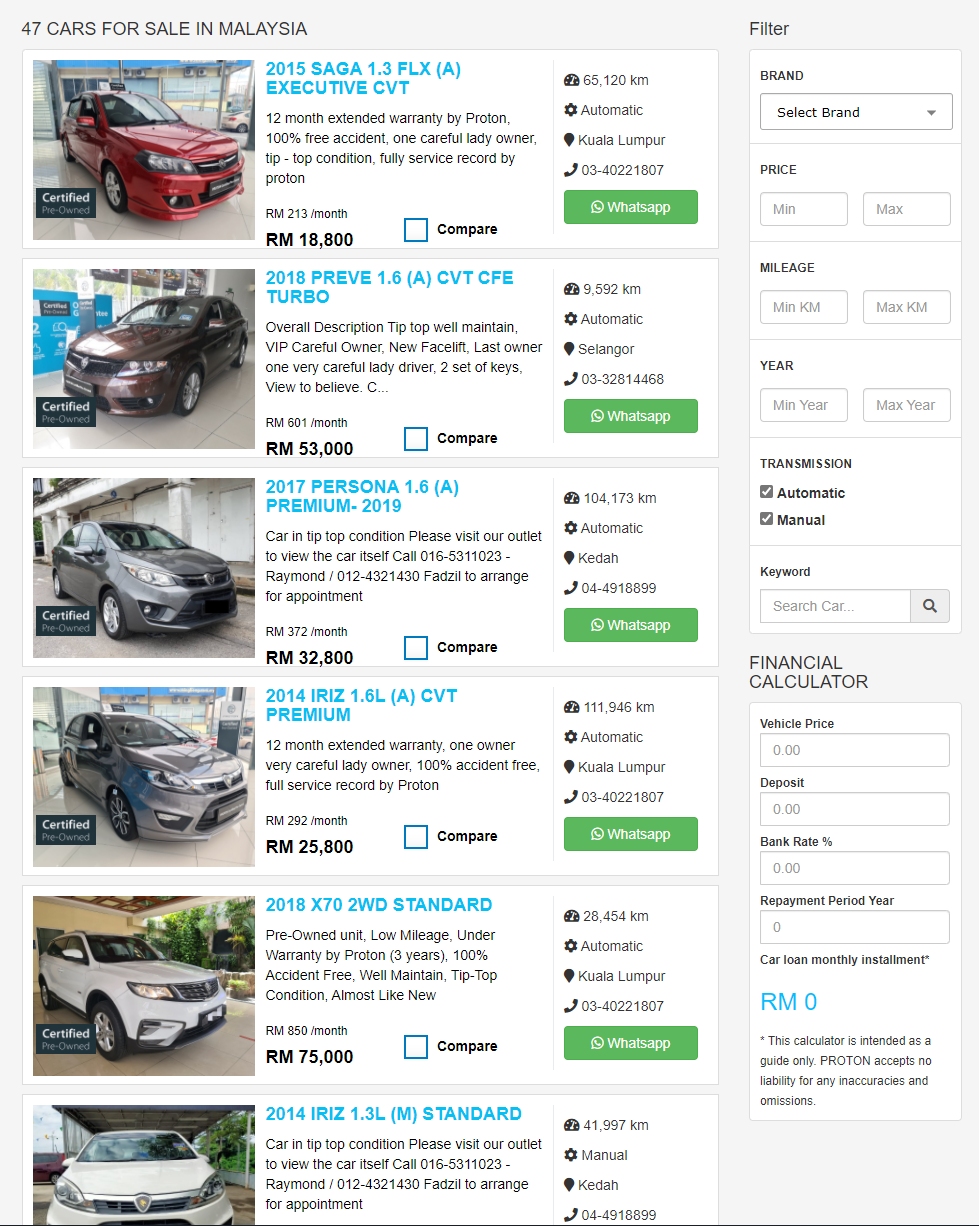The image features a light grey background with a header at the top stating, "47 cars for sale in Malaysia." Down the left-hand side of the image, there are six pictures of different cars, each accompanied by some details. Each listing includes the car model, a price (e.g., RM18,800 for the first car), and a blue outlined box that says "compare." 

Next to each car image is a series of icons on the right-hand side. Although the first icon is unclear, the second appears to be a gear shift, the third resembles a balloon or a map pin, and the fourth looks like a telephone. Below these icons is a green rectangle with "WhatsApp" written inside, recurrent in all the car listings.

On the right-hand side at the top, there is a filtering section. This section has a white rectangle labeled "Brand" followed by a grey outlined rectangle that says "Select brand" with a downward pointing arrow. Below that, there are filters for "Price," with two grey outlined rectangles labeled "min" and "max," and "Mileage," with two similar rectangles labeled "min KM" and "max KM." The "Year" filter also includes two grey outlined rectangles for "min year" and "max year."

The "Transmission" filter allows you to choose between "Automatic" and "Manual," each with checkboxes. Below this is a "Keywords" entry section with a grey-outlined rectangle and a magnifying glass icon within a grey square.

Lastly, there is a "Financial Calculator" section with white and grey-outlined rectangles for entering vehicle price, deposit, bank rate, and repayment period in years. The calculation result is displayed in blue as "RM0," with additional explanatory text in black following it.